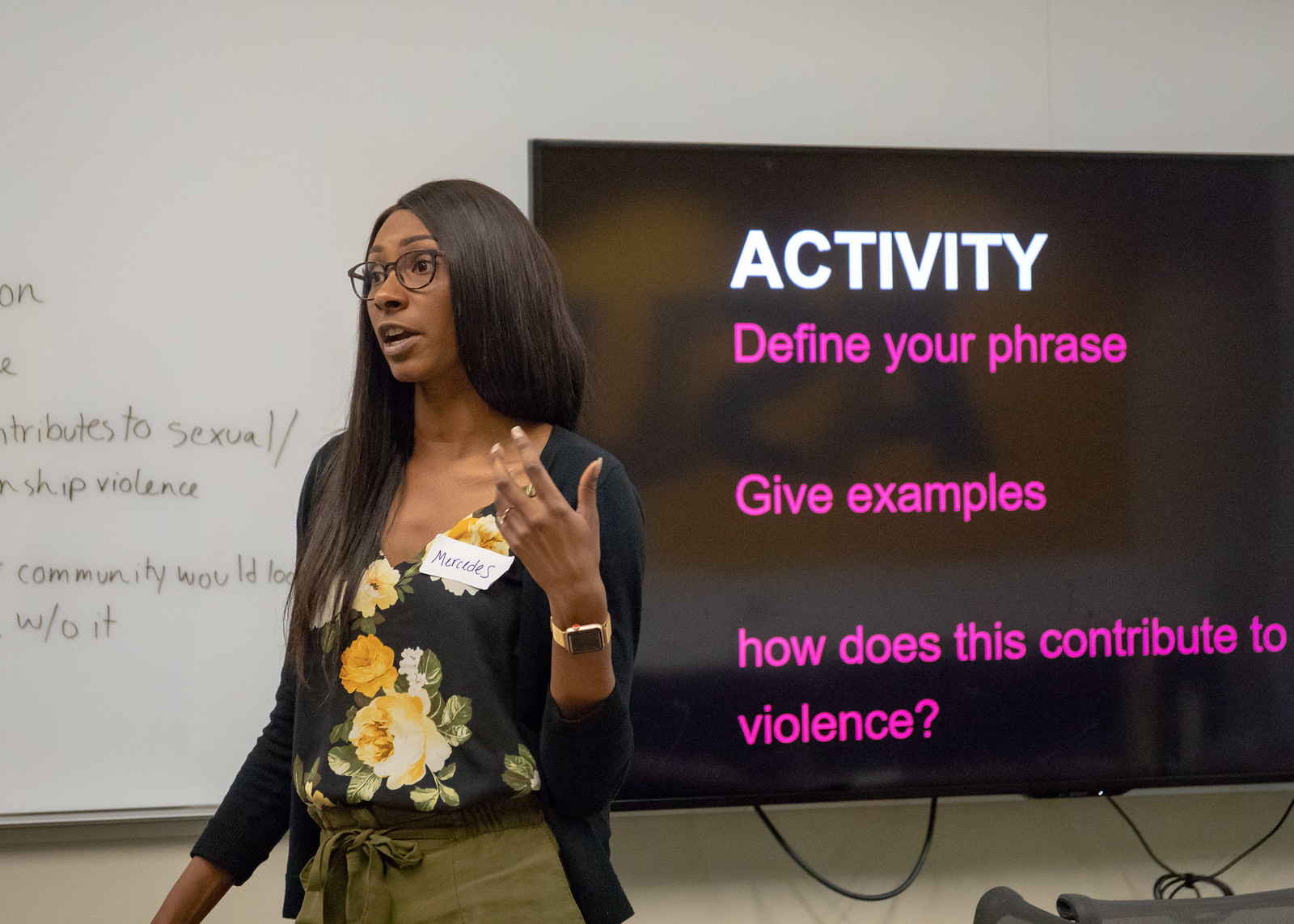The image shows a woman named Mercedes, who appears to be giving a lesson or presentation while standing in front of a large whiteboard and an even larger TV monitor. Mercedes has dark brown skin, long dark hair, and is wearing tortoiseshell glasses. She is dressed in a black blouse adorned with large yellow and white flowers, paired with a black cardigan. Her olive green pants tie at the front with a drawstring. She is also wearing a watch with a gold band and a black face on her left wrist. 

The TV monitor behind her displays a black background with white and pink text. At the top, in bold white letters, it reads "Activity." Beneath this, in pink text, it instructs, "Define your phrase," "Give examples," and asks, "How does this contribute to violence?" The whiteboard, partially visible to her right, has handwritten black text, some of which reads, "contributes to sexual/relationship violence, community," though much of it is cut off and not fully legible. Mercedes is gesturing with her left hand raised while her right hand rests at her side.